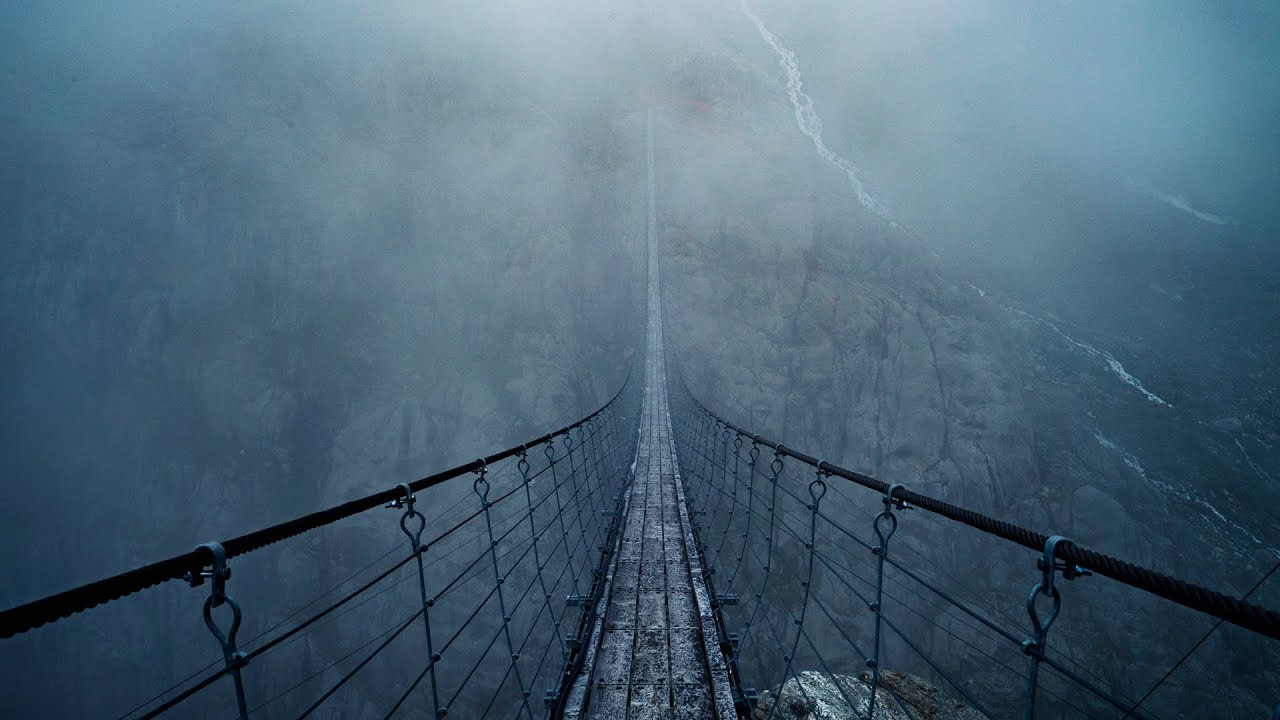Looking down from a dizzying height, this image captures a nerve-wracking view of a very long, high drawbridge suspended between two massive, rocky mountain peaks. The bridge, recalling scenes from movies that make your stomach churn, consists of three weathered wooden planks, bordered by black cables and wire netting that make up its delicate-looking railings. The boards are aged, with some moss growing on them, but all are intact. Enveloped in thick fog and mist, the scene is shrouded in an eerie, smoky atmosphere, suggesting that the bridge is nearly at cloud level. The mountains themselves are barely visible through the haze, though a large stream cascades down one side. The emptiness and the light's dimness add to the unsettling effect, making the bridge appear to sway and move with the wind, evoking a profound sense of vertigo just from the image alone.